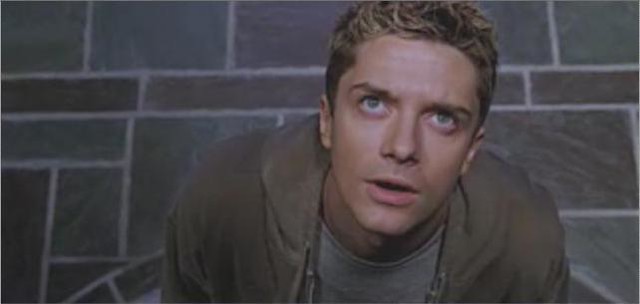The image depicts a young Caucasian male, who appears to be Topher Grace in his early to mid-20s. He has short blonde hair, slightly longer and styled on top with the sides cut close to his scalp, and blue eyes. He is clean-shaven, with reddish undertones beneath his eyes, suggesting he might be tired. Wearing a gray round neck shirt with a light brown or drab gray jacket layered over it, he is leaning slightly forward at the waist. The shot captures him from mid-chest to the top of his head as he looks upward to his right, seemingly focused on something to the left out of the camera's view. He stands in front of an irregularly patterned brick wall, consisting of gray and red bricks with visible mortar in between.